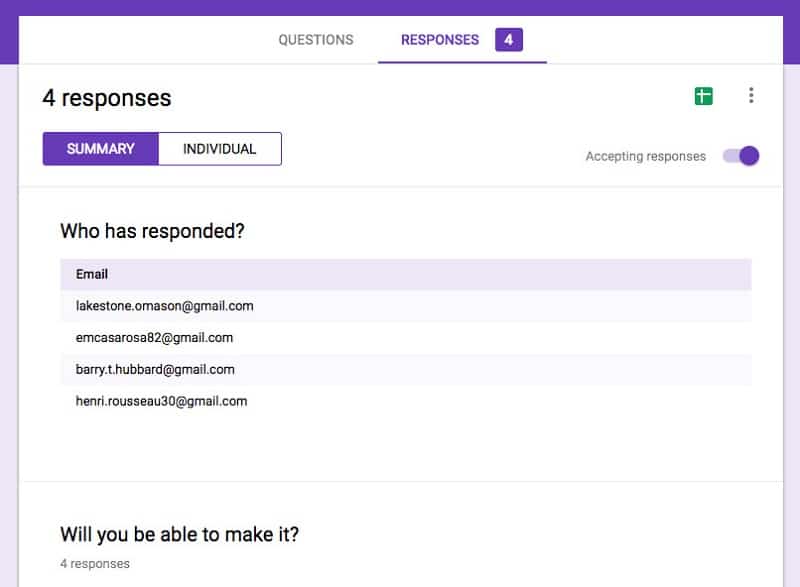This image is a screenshot from an unspecified digital source, focusing on a user interface related to gathering responses. At the top of the image, the heading "Questions" appears, followed by "Responses (4)", with the number "four" underlined by a thin purple horizontal line. The responses section features a tab labeled "Summary," which is currently selected, alongside another tab labeled "Individual." Underneath, the status "Accepting responses" is indicated with a slider button set to "On."

Following this setup, there is a prompt asking, "Who has responded?" Correspondingly, there are four listed email addresses of respondents: blakestone.omason@gmail.com, emcasarosa82@gmail.com, barry.t.hubbard@gmail.com, and onry.russo30@gmail.com. Another prompt appears asking, "Will you be able to make it?".

The image is enclosed by a border that is pale purple up until the top corners and edge, where it transitions into a darker shade of purple. It should be noted that additional text is slightly visible but cut off at the bottom of the screenshot. This lower section does not feature a border. The screenshot exclusively showcases textual information and interface elements, devoid of any photographic content, people, animals, plants, buildings, or automobiles.